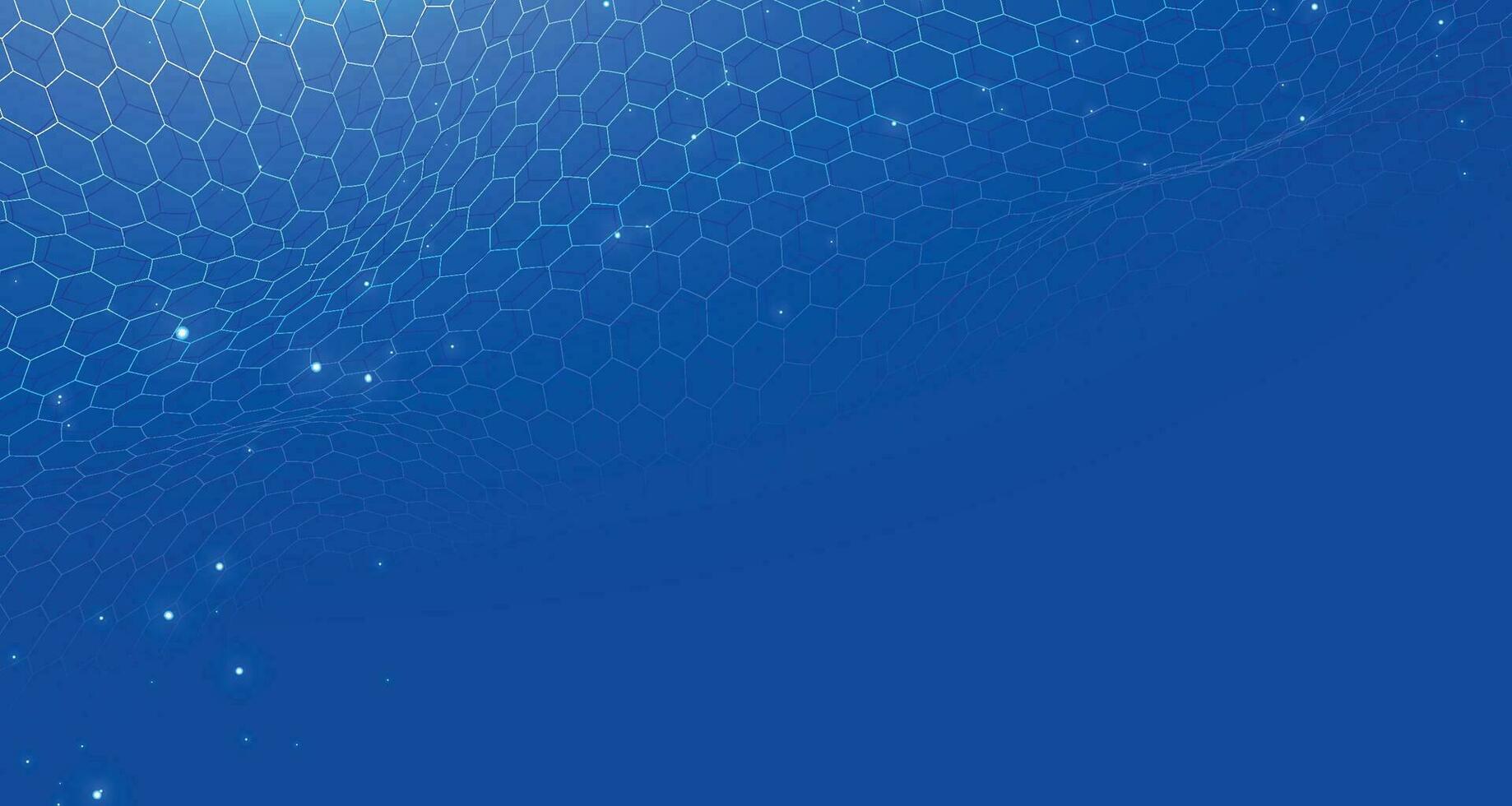This calming, AI-generated image features a gradient of blue hues, ranging from a clear indigo at the bottom to an aqua blue at the top. It is dominated by a hexagonal pattern that emerges most prominently in the top left corner. These hexagons are outlined in white and interspersed across the top portion of the image, with a subtle duplicate pattern visible in black behind them. The pattern of hexagons gradually fades as it moves downwards, blending smoothly into the blue background. Scattered throughout the lower left corner and extending towards the center are small, glowing white dots, reminiscent of stars, adding a sense of depth and tranquility to the image. The overall effect is a harmoniously structured, yet soothing visual experience, akin to looking through a watery substrate at a softly illuminated honeycomb.